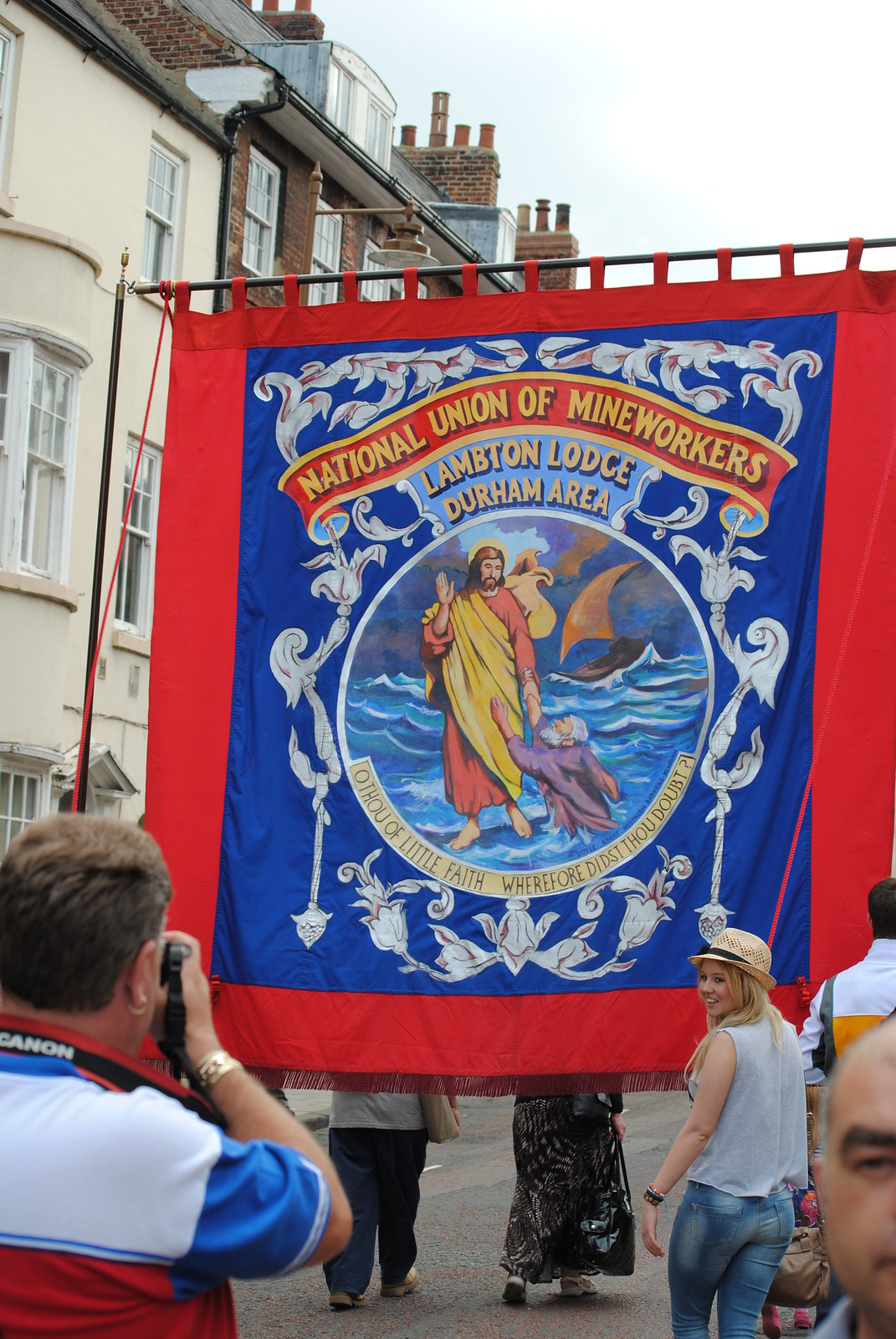In this vividly detailed outdoor photograph, a group of people is depicted walking down a street during what appears to be a parade. Central to the image is a prominent banner held up by poles, which is adorned with striking red borders and a vibrant blue center. The banner features an intricate design, including a gold-trimmed red ribbon with the words "National Union of Mine Workers" inscribed across it in gold text, and beneath that, "Lambton Lodge, Durham Area" is similarly inscribed. The focal point of the banner is a depiction of a bearded figure, reminiscent of Jesus, dressed in a red robe with a thick gold sash over his right shoulder. This figure appears to be walking on water, extending a hand to aid a man who is half-submerged, seemingly in distress, dressed in purple with grey hair and a beard. Surrounding the banner, there are several individuals with their backs turned to the camera, contributing to the sense of movement and action. Additional details include buildings on the left side of the street, and a serene sky above, painted in hues of blue and white. In the crowd, specific people stand out, such as a heavyset man in a red shirt taking a picture, a blonde woman in a hat wearing a white top and blue jeans, and various others, some dressed in black pants and white shirts, enhancing the rich narrative of the scene.